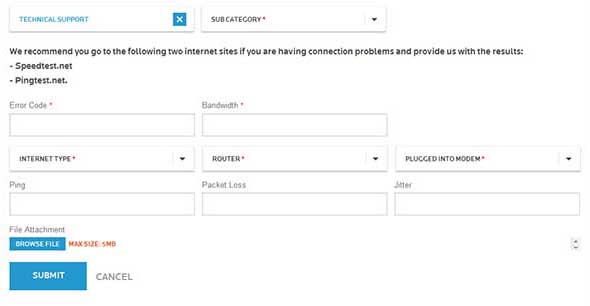The image features a white background with multiple sections dedicated to technical support instructions. At the top, there's a header box labeled "Technical Support" that includes a teal square with a white 'X' inside it.

Below this header is a subcategory box marked with a red star, indicating mandatory fields. Directly underneath, there is a message in black text advising users to visit two specific internet sites if they encounter connection problems and to provide the results. The recommended websites are listed as:
- Speedtest.net
- Pingtest.net

Following this, there is a series of labeled fields and input boxes:

- "Error Code" (marked with a red star) with a black outlined box for inputting the code.
- "Bandwidth" (marked with a red star) with a matching box for entry.
- "Internet Type" (marked with a red star).
- "Router" (marked with a red star).
- "Plug into a Modem" (marked with a red star).

In the next row on the left side, the labels include:
- "Bing" with a grey-outlined input box.
- "Packet Loss," also with a grey-outlined box.
- "Jitter" (though this part of the image is blurry).

At the bottom, there's a section for file attachments featuring two teal-colored rectangles. The first rectangle, labeled "Browse File" in white text, allows users to select files. The second rectangle, also with white text, is labeled "Submit" for submitting the attachment.

Each element is clearly distinguished and structured to guide users through troubleshooting and reporting their internet connection issues clearly and effectively.